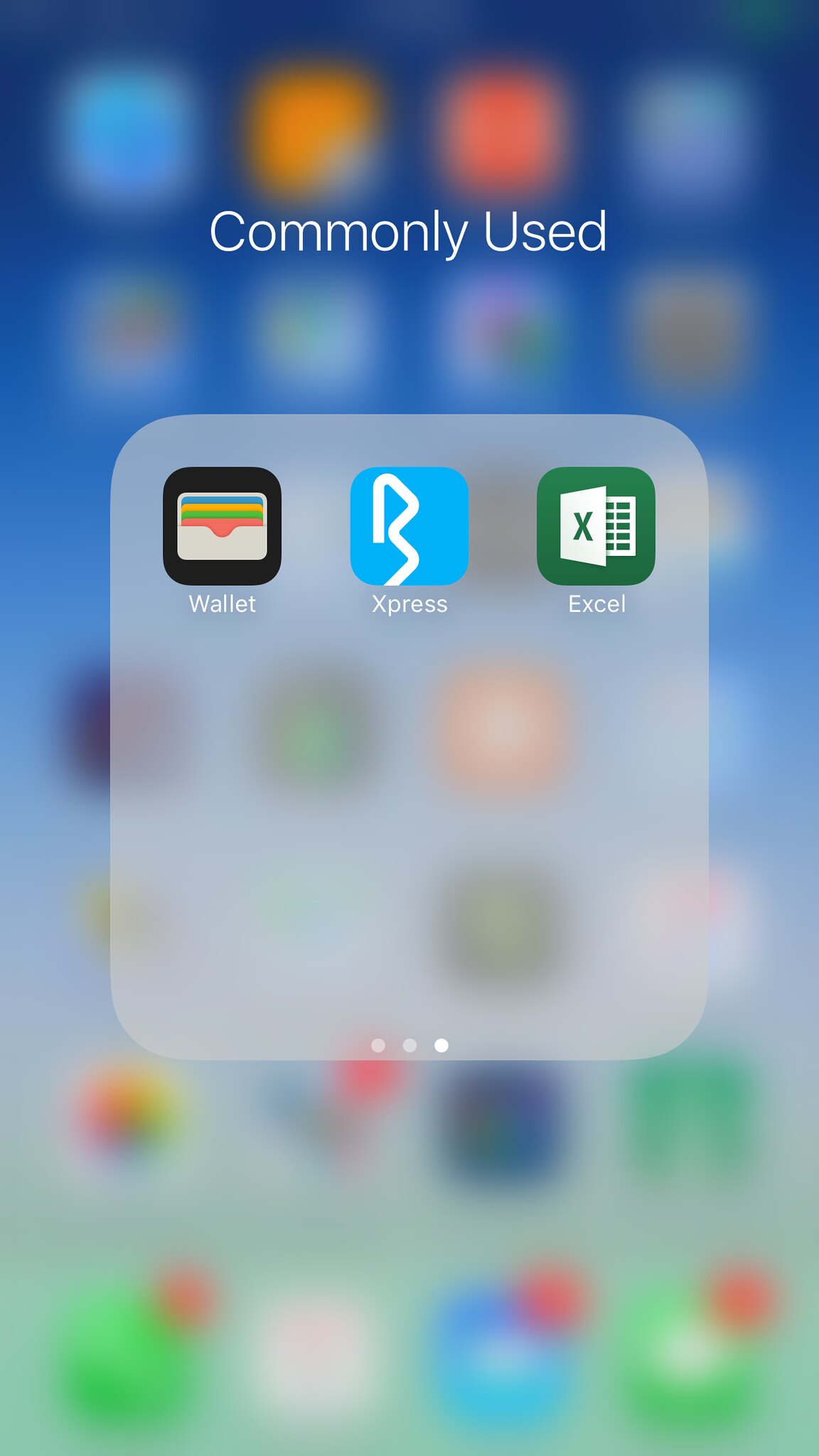The image features an iPhone with a variety of app icons displayed on a predominantly blue background, which transitions to white near the bottom. Most of the app icons are intentionally blurred, making them difficult to identify. However, some details can still be discerned. 

At the bottom of the screen, there is a clear, unblurred section showing a few commonly used apps. The caption "commonly used" is displayed in a moderate white font above the icons. Among the clear icons are Wallet, Express, and Excel.

- **Wallet**: The icon depicts a stylized wallet containing various cards.
- **Express**: This app is represented by a blue square with a white, squiggly line.
- **Excel**: The familiar green icon of Microsoft's Excel app, featuring a white file sheet with a large "X" on it.

Additionally, some of the blurred icons at the bottom show notification indicators. For instance:
- A green phone icon with a red notification badge, suggesting a missed call.
- A green text message icon with a white speech bubble and a red notification badge, indicating unread messages.
- A potential photo app icon above the phone icon, featuring a cloud.

While the image primarily emphasizes the three commonly used apps with clear icons, it also subtly illustrates the presence of other applications and notifications on the iPhone's home screen.